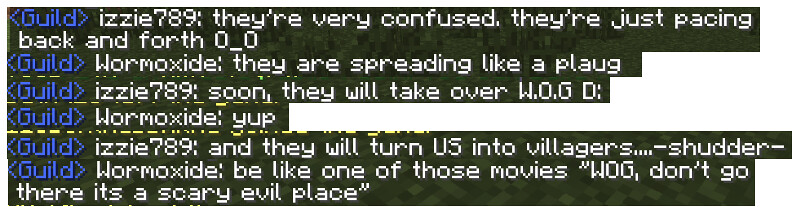The image is a long, narrow, almost rectangular screenshot of a conversation between video game players on a computer. The conversation is presented in a series of green text boxes cropped to the length of the sentences, set against a white background. On the far left, each line begins with the word "Guild" inside blue arrows. Following the word "Guild," the speaker's username appears in white text. 

The dialogue unfolds as follows: Izzy789 expresses confusion, stating they are pacing back and forth, accompanied by the wide-eyed emoticon "0_0." Wormoxide responds next, mistakenly typing "plaug" instead of "plague," indicating something is spreading rapidly. Izzy789 then mentions that soon there will be a takeover involving "W.O.G," followed by a capital "G" and a colon. Wormoxide replies with a simple "yep." Izzy789 adds a dramatic note about being turned into villagers, using ellipses and dashes to emphasize the shutter effect. Finally, Wormoxide compares the situation to a scary movie, cautioning against going to the place referred to as "W.O.G."

This detailed exchange highlights a sense of urgency and confusion, underscored by the use of emoticons, misspellings, and dramatic punctuation.